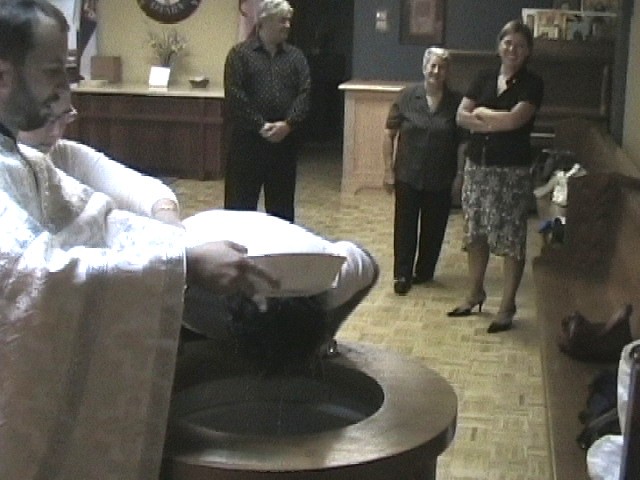The image captures a baptism ceremony, seemingly held in a church setting but the low resolution suggests it was taken with older technology. On the left, a priest dressed in white vestments with a beard and partially balding hair, pours water from a white bowl onto the head of a person leaning over a baptismal font. The font has a circular opening filled with water. The person being baptized wears a white shirt and is bent over the font, receiving the sacrament. In the background, three onlookers are smiling—a man in a black long-sleeve shirt and black pants stands in the center, flanked by two women. One woman wears a skirt and black shirt with crossed arms, and the other also dressed in black, with a button-down shirt and pants. The scene is framed with church pews, indicating additional religious context and suggesting multiple baptisms may have occurred.